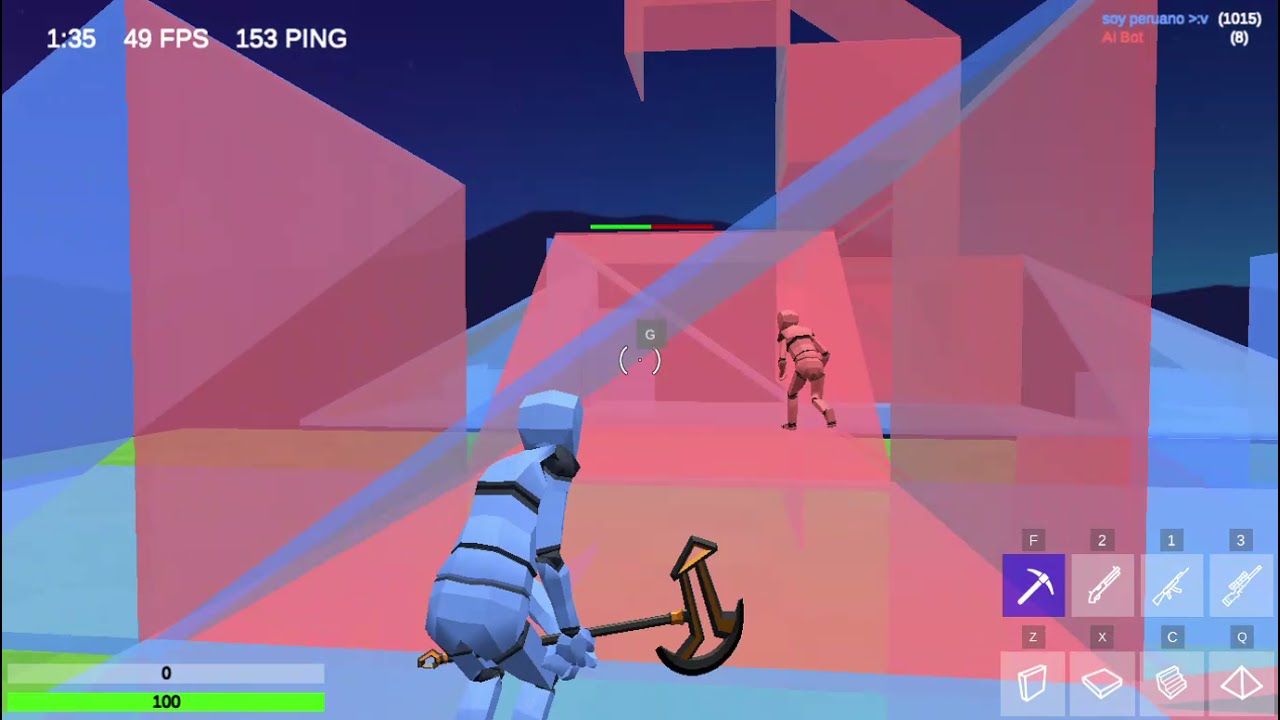In this detailed screenshot from a video game, likely Fortnite, the scene showcases a robotic character equipped with white, banded armor reminiscent of a stormtrooper, crouched and holding a unique weapon resembling an axe. The axe features a long pole with a curved piece of metal at the end, adorned with twin prongs and a triangular extension, suggesting a specialized tool or weapon. The robot's stance indicates readiness, with knees bent and arms gripping the axe as if preparing to engage an unseen adversary in the distance.

In the environment, there are both transparent cube walls and vividly colored pink and blue geometric shapes, creating an abstract battlefield. Another player, dressed in similar white armor, is seen in the background, possibly being pursued. The bottom left corner displays a dual-status bar with a zero marker and a fully green 100% marker. A weapon grid is present at the bottom right, showcasing various weapons including the equipped pickaxe and multiple firearms, totaling eight inventory items.

The top of the screen reveals game performance metrics: 49 fps (frames per second) and a ping of 153. Additional information displays time-related data, with "10:15" in parentheses and the number "8" below it. The overall scene underlines a fast-paced, tactical environment with meticulous attention to character and weapon details within a vibrant and dynamic game space.